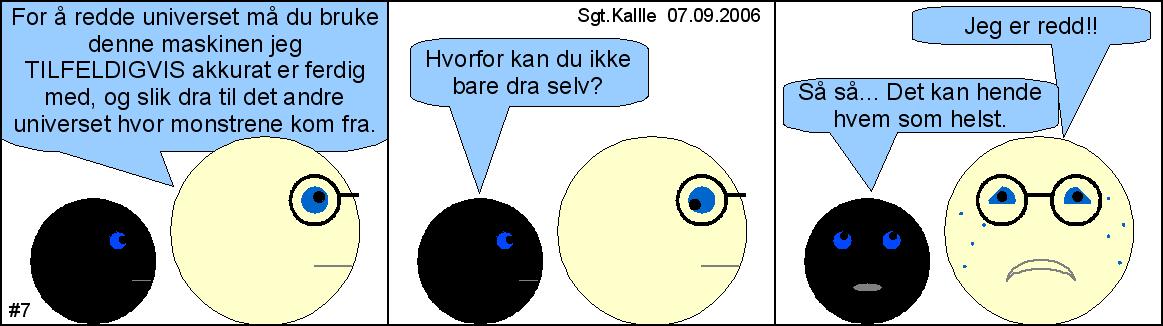The image is a digitally drawn, three-panel comic strip created with a primitive computer program. Each panel has a white background and black borders, and is structured with simple circles for characters. In the bottom-left corner of the comic, the number "7" is inscribed. Additionally, the top of the strip features the text "Sgt. Calais, 07-09-2006".

In the first panel, a small black circle with a blue eye and a larger yellowish circle, also with a blue eye but wearing black glasses, face to the right. The larger circle speaks first, with a blue speech bubble containing text in what appears to be German.

In the second panel, the setup remains the same except the positions of the speakers switch: the black circle now speaks while the yellow circle looks at it, featuring another blue speech bubble filled with text in the same foreign language.

In the third and final panel, both circles face directly forward. The yellow circle appears sad, with drooped lips and tearful eyes, suggesting a state of despair. The black circle looks towards it, possibly in a moment of sympathy or consolation. Blue speech bubbles above each character contain the phrases "Sasa.com" from the black circle and "Jagger Red" from the yellow one.